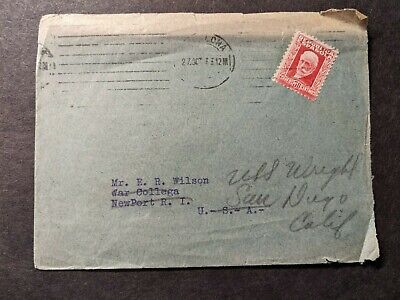This detailed photograph showcases a vintage envelope sitting on a weathered wooden table. The envelope itself exhibits signs of age, with a faded blue color on the front and a top edge that has become almost pinkish over time. In the upper right corner of the envelope, there is a red postage stamp featuring an older man with white hair and a beard, placed diagonally with the bottom left tilted upwards. The central portion of the envelope includes a partially legible circular stamp, displaying the letters "O-N-A" at the top. Additionally, there’s a mix of typed and handwritten inscriptions on the envelope. The typed address reads "Mr. K. R. Wilson, Collega, Newport, RI, USA," although much of it is struck through. Adjacent to this is cursive writing that states "ULD Wright, San, New, California." The photo’s backdrop is dark and unobtrusive, emphasizing the weathered envelope and its historical essence.